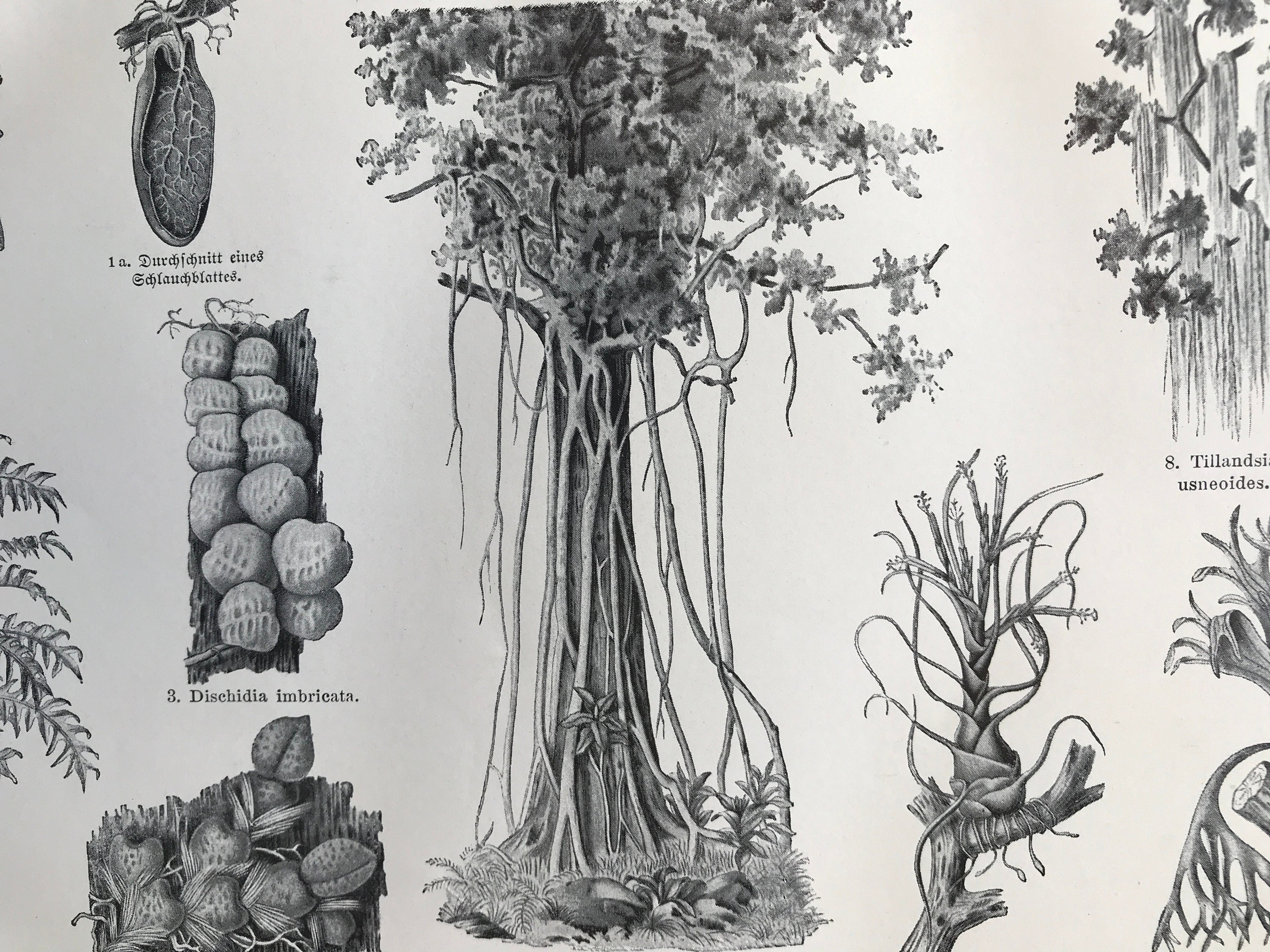The image is a clear, black-and-white pencil drawing that appears to be a digital scan of a book page, featuring detailed illustrations of various plants and trees, with an emphasis on botanical elements and wildlife. The background is a light gray, resembling a page in a book, and the image is divided into distinct sections labeled with numbers and captions in a non-English language.

In the top left corner, there is a peculiar illustration that resembles a large, meaty leaf with prominent veins, somewhat akin to an internal human organ. This is labeled with "1A Durdenit Ains Edlan Blottes." Below this, there are two neat rows of what look like peanuts trapped in a shell, organized into six columns, and labeled "3. Dischidia imbricata."

A large central image dominates the middle, displaying a vertically oriented tree with its branches and leaves spread out at the top, giving an impression of a bird’s nest with baby birds. Branches are drawn vertically, adding to the detailed depiction.

On the right-hand side, labeled with the number eight, there are additional illustrations of leaves and branches. The drawing is meticulously detailed, providing clear visual information despite the language barrier in the text descriptions.

Overall, the image captures various parts of trees, such as leaves, branches, and nuts, in a well-lit and clearly visible setting, with each section carefully labeled and illustrated.